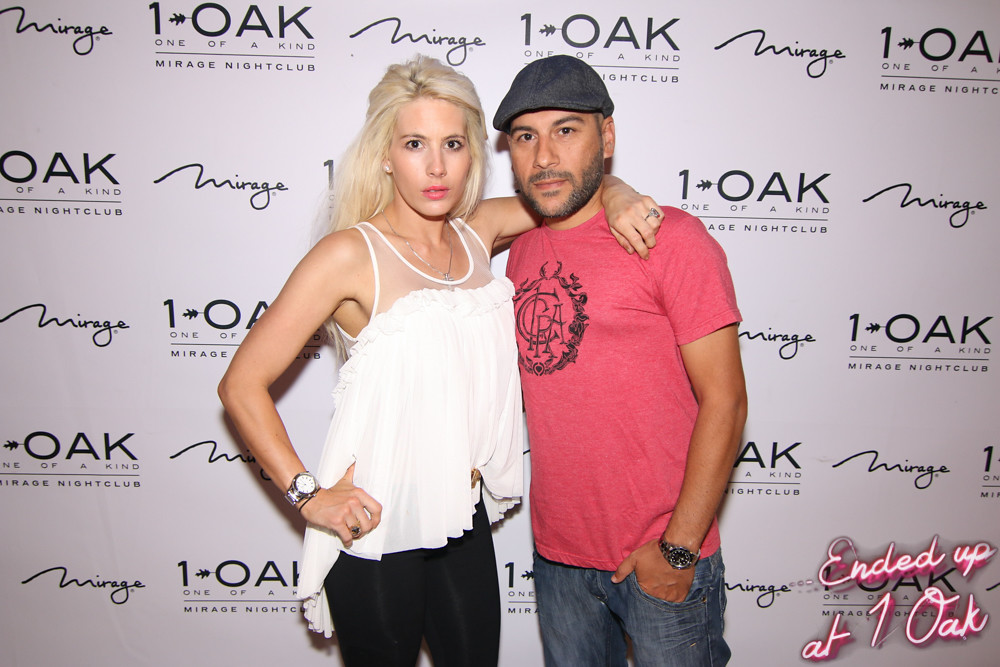A photo captures a casually dressed man and woman at a red carpet event in front of a promotional backdrop adorned with repeating logos of "One Oak" and "Mirage Nightclub." The woman, positioned on the left, is a blonde with dark brown eyes, dressed in a distinctive white tank top with sheer straps and a flowing fabric below the chest, paired with black pants. The man, standing to her right, wears a blue English cap and a red t-shirt featuring a design that reads "CCRA" with a laurel motif. He pairs this with blue jeans and a wristwatch. The backdrop behind them features rows of the "One Oak" and "Mirage Nightclub" logos, and in the bottom right corner, the phrase "Ended Up at One Oak" is prominently displayed in white text with red accents.